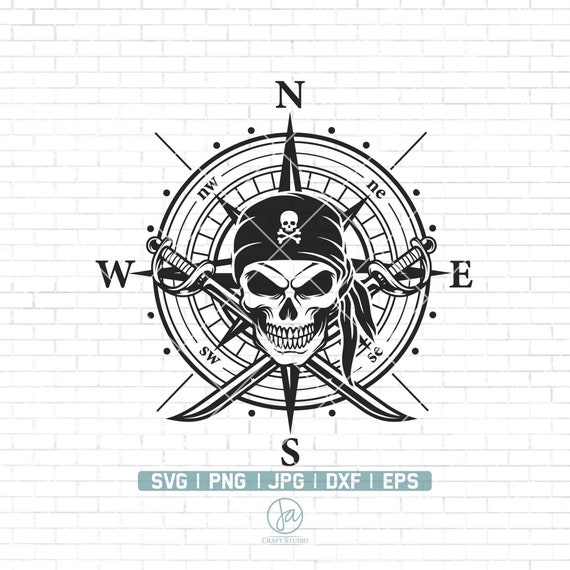The image is a detailed and finely graphic representation that combines elements of classic pirates and navigational symbols, plastered against a simulated white brick wall backdrop, which looks reminiscent of subway tiling with gray outlining. Central to the image is a meticulously designed black-and-white compass adorned with a smiling skull, more cheerful than menacing, replacing the typical crossbones with crossed swords. Each cardinal and intercardinal direction—North, South, East, West, Northeast, Northwest, Southeast, Southwest—is clearly marked with sharp arrow tips. A touch of craftsmanship is evident in the minor detailing, such as dots flanking each directional letter. Underneath the compass is a blue box displaying text in white letters, listing five different file formats: SVG, PNG, JPG, DXF, and EPS. Additionally, a logo featuring the lowercase letters "j" and "a" within a circle, followed by the phrase "Craft Studio," is present, indicating the creative source of the artwork.